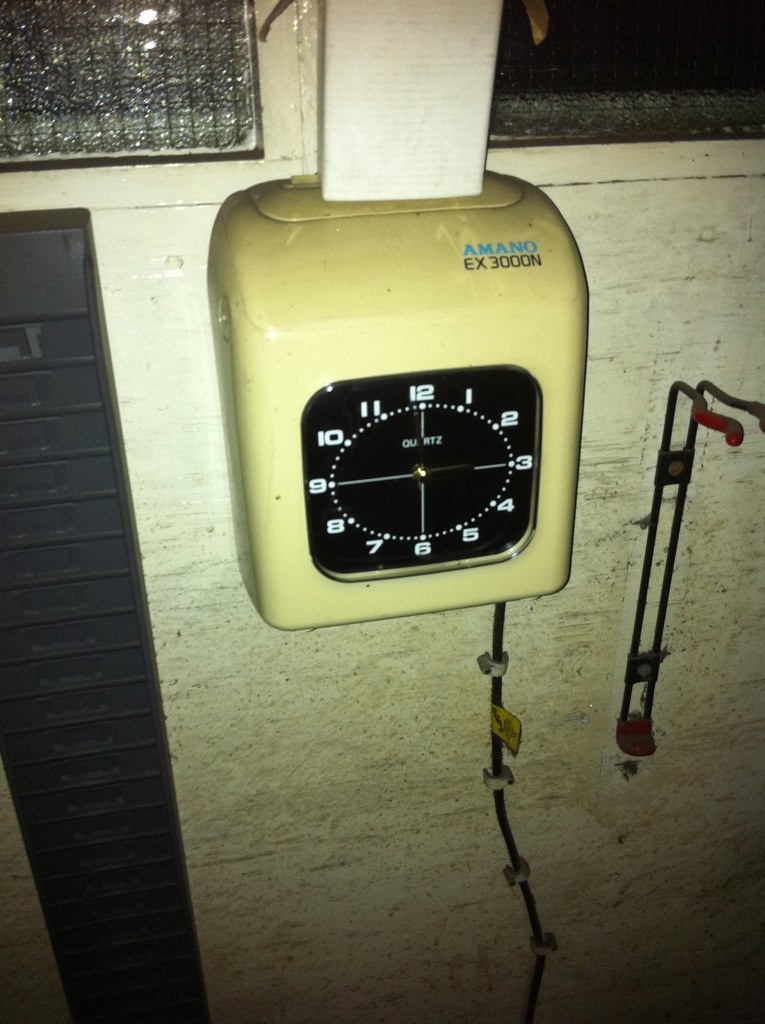The image depicts an old-fashioned Amano EX3000N time clock, mounted on a somewhat dirty, textured beige wall with a pale yellow hue. The wall also features the right bottom corner of a glass window with vertical black lines. The time clock, distinct with its yellowish color—likely from age and lack of upkeep—features a black clock face with a white numerical dial arranged from 1 to 12 and white clock hands indicating hours and minutes but no seconds. Mounted to the left of the clock is a plastic rack intended for holding time cards. A power cord is visibly tacked to the wall, running down from the bottom right of the time clock.